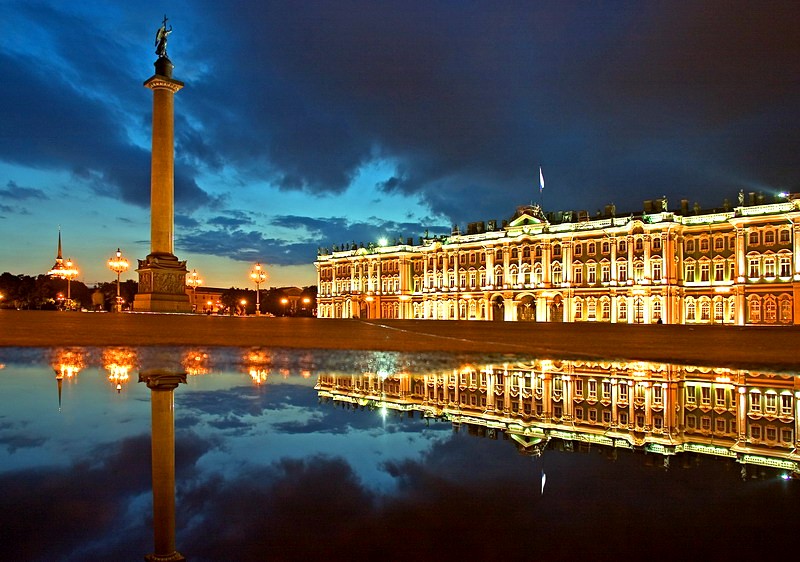This image captures a magnificently illuminated historical building in St. Petersburg, Russia, taken during late evening or night. The large white palace stands prominently on the right, bathed in a bright yellow-gold light, with intricate architectural details reflected perfectly in the smooth, still water of a man-made pond below it. This reflection creates a stunning mirrored image of the building, the sky, and surrounding elements. To the left, a grand statue, possibly an angel holding a cross, towers on a white marble base and pole, facing the palace. Streetlights, signage, and a distant steeple or tall tower structure add to the scene’s depth. The navy blue sky is tinged with shades of blue and a hint of yellow near the horizon, suggesting either sunset or the glow of city lights. The peaceful ambiance is accentuated by spotlight beams illuminating a flag atop the palace, and the scene is framed with a fence around the water, giving the photo a balanced and majestic composition.